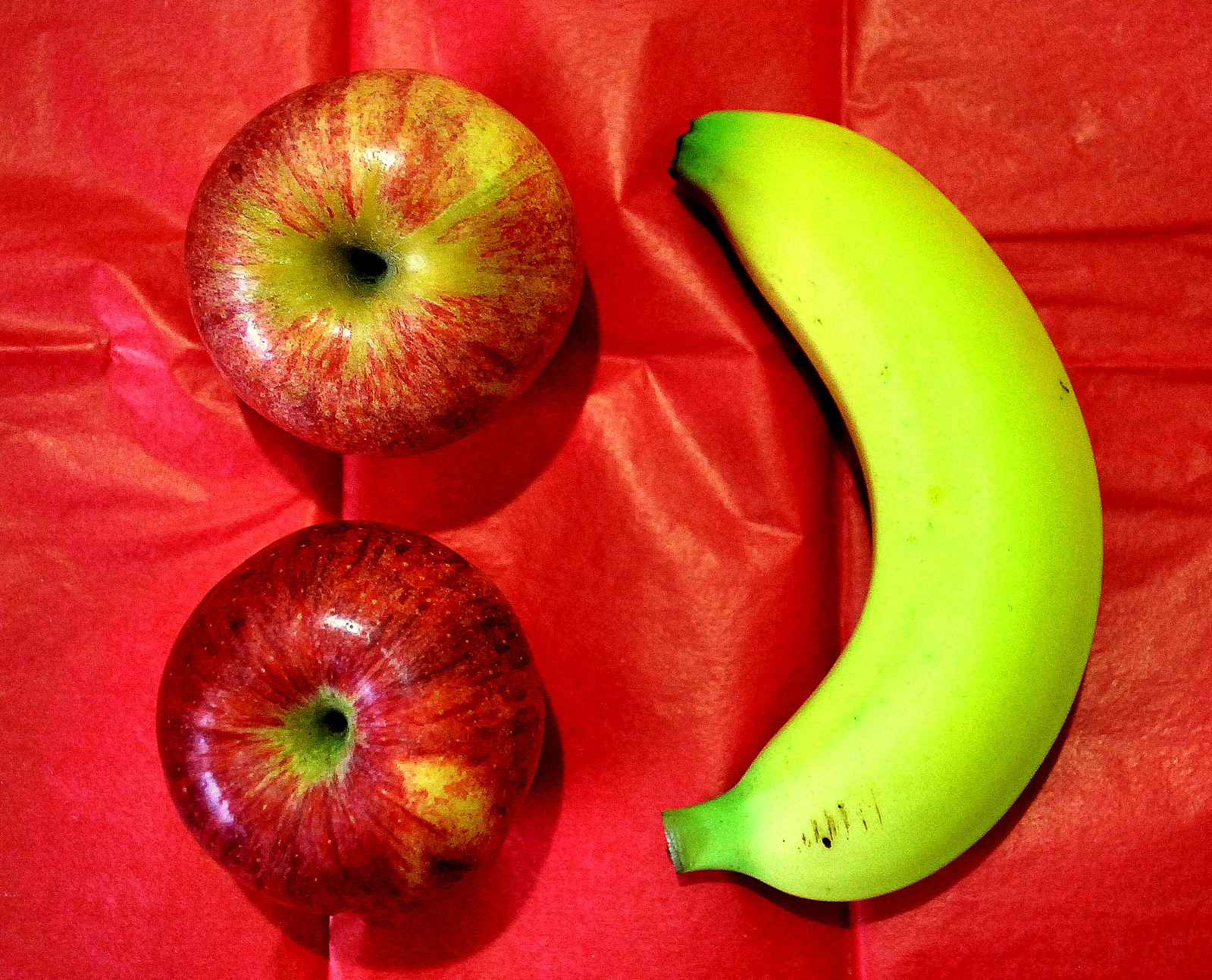A vibrant still-life image showcases two red apples and a single banana arranged on a rich red fabric, viewed from directly above. The two apples, featuring subtle green bursts around their stem areas and marked with streaks of darker red, are positioned on the left side of the scene. They are aligned vertically in a neat column, sitting firmly on their bottoms. To the right of the apples, a plump banana with a slightly green tip and stem lies almost alongside them, also in a vertical orientation. The banana curves naturally, occupying as much vertical space as the two apples combined. The red fabric beneath them is slightly wrinkled, adding texture and contrast to the composition. The entire arrangement creates a harmonious and visually appealing still life, inviting viewers to observe the intricate details and colors of the fruit.